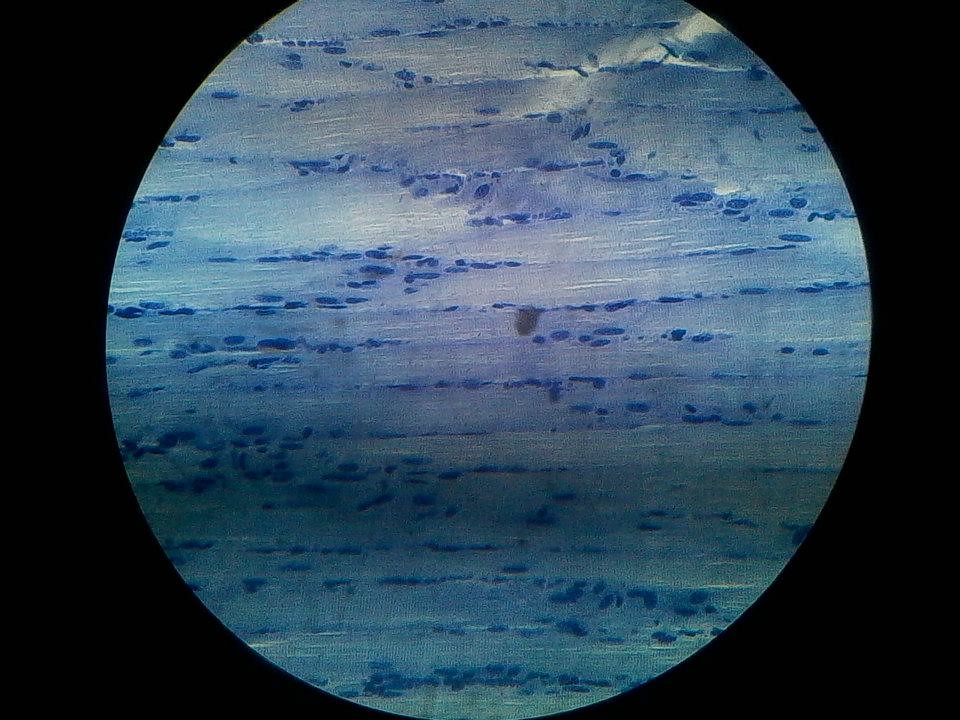This microscopic image captures a detailed view of a gray surface, which could likely be skin or wood grain. The surface shows intricate patterns with light gray tones interspersed with round, darker blue cells reminiscent of corpuscles. These blue cells mostly align in linear formations, except at the very bottom, where they cluster more densely and appear darker. The image also reveals white and light blue streaks or striations throughout, contributing to its textured appearance. Towards the center, a small brown spot is visible, possibly a blemish on the lens or the surface itself. Additionally, a subtle light green tinge appears at the bottom of the frame. The upper right corner of the image shows some distortion, giving a prism-like effect, adding a unique dimension to the overall composition. The viewing area is circular, accentuating the meticulous details and varied textures captured by the microscope.